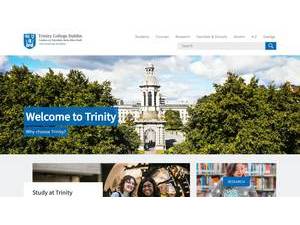The website features a welcoming section presented in a blue rectangle with the text "Welcome to Trinity" in white letters. Beneath this, another blue rectangle contains the phrase "Why Choose Trinity", indicating that the website pertains to a college. Despite the small text size at the top, it is distinguished by five words and includes a search section. This section is marked by a gray rectangle with the word "Search" inside, accompanied by a blue square with a white magnifying glass icon.

The central image showcases a large college building surrounded by numerous trees, under a sky filled with white clouds and light blue hues. Below this image, three distinct sections are displayed. 

The first square highlights the phrase "Study at Trinity", reinforcing the academic nature of the institution. The second square features an image of two smiling girls, presenting a friendly and welcoming environment. The third square depicts a woman in a library, with numerous books visible in the background, suggesting academic resources and support. Text is displayed across part of this picture, adding further context.